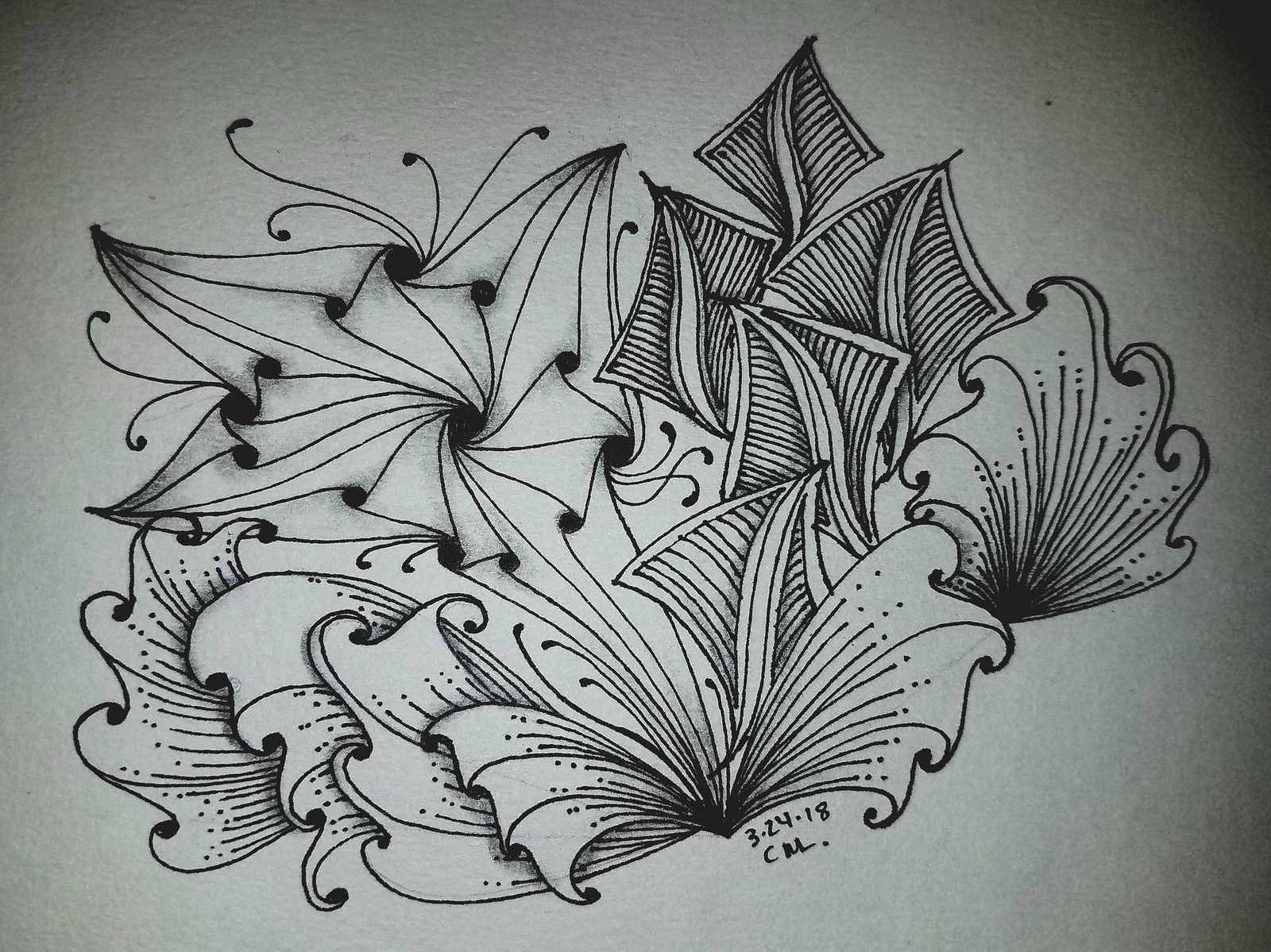This black ink drawing, resembling a zentangle artwork, is set against a stark white background with subtle black shadows in each corner, giving it a framed appearance. The piece features intricate, abstract patterns that suggest the shapes of flowers and leaves. At the bottom, a prominent flower extends its patterned leaves to the left and right, creating a repetitive and harmonious design. Above the leaves, triangular shapes resembling sails are integrated into the composition, lending a dynamic flow to the piece. On the upper part of the drawing, a pinwheel-like pattern with repeated angles forms, enhancing the overall mesmerizing effect of the artwork. Long, squiggly lines with dots at their ends and kite-like shapes with stripes intricately weave through the abstract floral and leafy elements. The drawing is dated 3-24-18 and signed with the initials CM, although another account mentions the initials as C, N, L. The high-quality photograph captures every detail of the meticulous line work, making it possible to appreciate the complexity and finesse of the design.